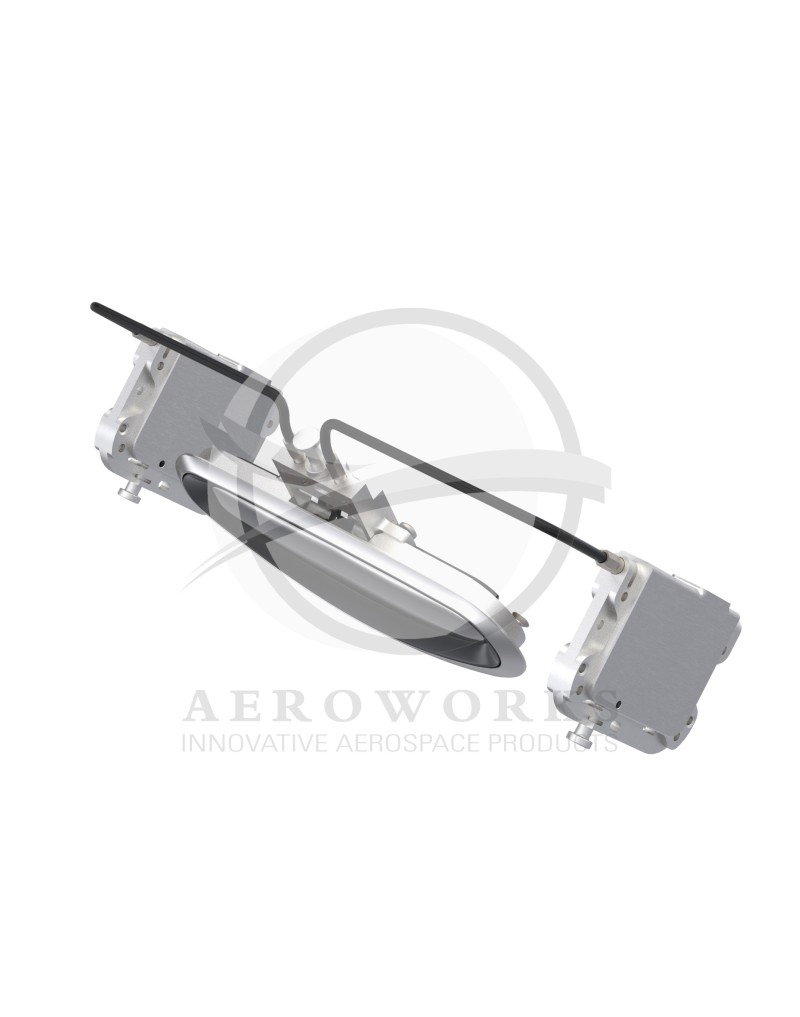The black and white image appears to be an advertisement for a company named AeroWork, specializing in innovative aerospace products. The main focus is a metallic device of undetermined function, likely used in aerospace construction. This device is centrally located and features a complex structure: two thin, black arms extend from a central, rounded component and connect to square-shaped metal pieces on either side. An oval-like element, reminiscent of a mirror but not reflective, is also part of the assembly. The background is solid white, and there is a light gray, semi-transparent watermark displaying the text "AeroWork Innovative Aerospace Products" in capital letters, with "AeroWork" in a larger font. Above the text is a distinctive logo consisting of a gray circle intersected by a brush-stroke-like line, resembling a blade of grass angled from the middle right to the lower left.